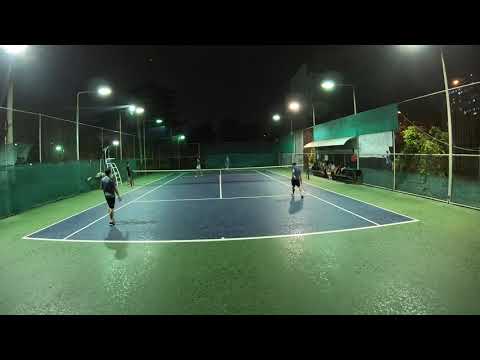The image portrays a nighttime scene of a tennis court, characterized by its distinctive design and illumination. The court features a dark blue playing surface with white lines, set against a lime green border. The view is slightly distorted due to a fisheye lens effect, with black bars occupying the top and bottom eighths of the photo. Central to the picture, a doubles match is in progress, with four players—two on each side of the net. The two players close to the foreground are wearing black pants and dark blue shirts; they both have short black hair. On the far side of the court, two more players are seen, though their details are less distinguishable. The entire court is enclosed by tall chain-link fencing, with parts of the lower sections covered by green tarp. Multiple banks of lights are positioned along the fences, with six to eight lights each fully illuminating the court, revealing a dark, starless sky above. A bench area with a steel overhang is discernible on the right-hand side of the image. The net in the center and the overall setup confirm that this is a tennis court, though it could be mistaken for a pickleball court.